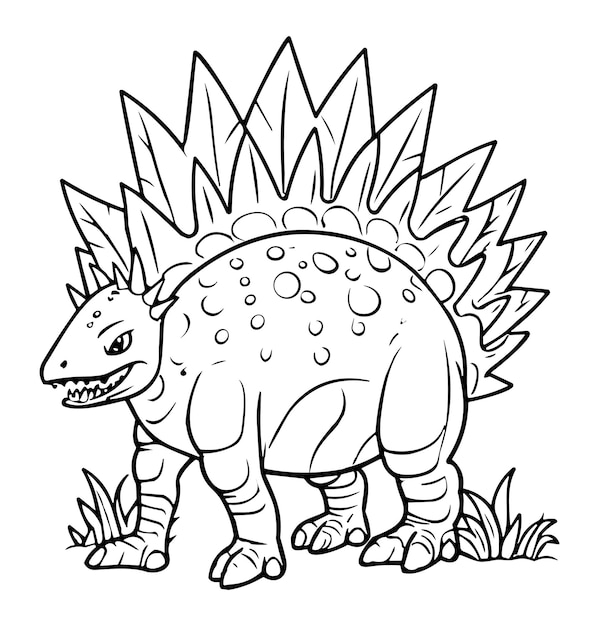This black and white digital drawing depicts a Stegosaurus, reminiscent of illustrations found in children's coloring books. The Stegosaurus is drawn with thick lines and appears to be facing the left, captured in a walking motion with its front left leg slightly back and front right leg forward. It has an intimidating expression with an open mouth revealing sharp teeth and a visible left eye. The head is adorned with six conical shapes, and the back features two rows of large triangular spikes that curve along its length, interspersed with smaller circles below the spikes and on its head. Each foot is rendered with three toes, and the dinosaur's two back legs are parallel. The ground beneath the Stegosaurus is dotted with small blades of grass on both the left and right sides of the drawing. The background is completely white, highlighting the details of this menacing yet playful prehistoric creature.